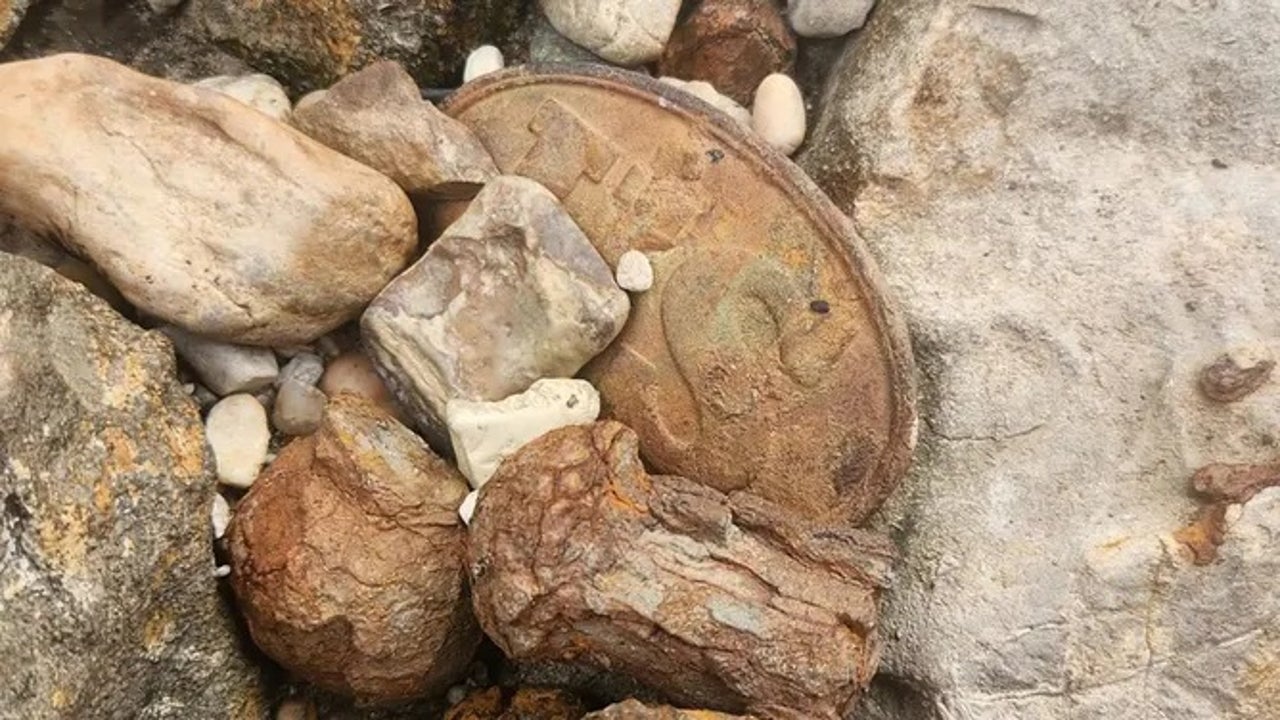This photograph captures a meticulously detailed scene of an antique Civil War-era U.S. Confederate belt buckle, heavily aged and weathered to a rusty patina. The oval-shaped belt buckle, with a raised edge and stamped with the capital letters "U.S.," is strategically nestled among an assortment of rocks. Positioned at a 45-degree angle with the left side pointing towards the top left corner, the buckle partially overlaps a large gray rock on its right side. A mushroom-shaped rock, bearing various shades of brown, lies sideways in front of the buckle, while a square gray mottled rock rests in front of the "U." Surrounding the buckle is a spectrum of rocks: one below the gray square rock is brown; another in the left-hand corner shows gray with light yellow and white hues; and above it, a smooth rock with light brown and tan tones partially overlaps the buckle. In the background, smaller multicolored rocks in shades of white, brown, and gray add further depth and texture to this historical vignette.